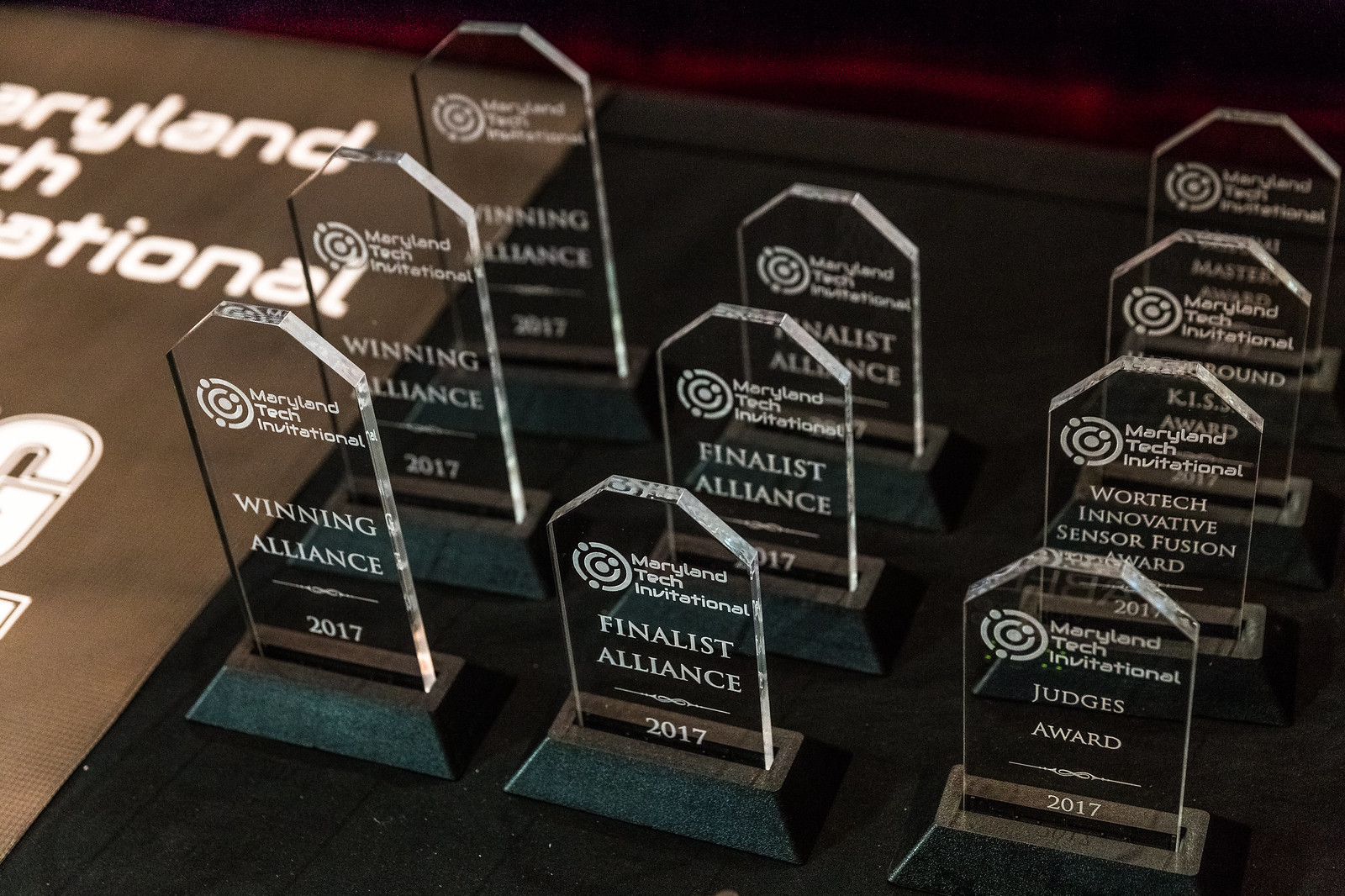This image depicts a black tabletop adorned with a series of glass awards arrayed in three distinct columns. Each award boasts a clear, tombstone-like shape with white etchings. Along the left side of the tabletop, partial text reads “Maryland Tech Invitational.” Adjacent to this text, the leftmost column features three “Winning Alliance” awards from the Maryland Tech Invitational, each bearing the year 2017 and standing on black bases. The central column consists of three slightly shorter awards also from the Maryland Tech Invitational, labeled “Finalist Alliance” with the year 2017 inscribed beneath. The rightmost column contains four awards. The front-most is distinctly marked as the “Judges Award 2017,” while another reads “Wartec Innovative Sensor Fusion Award 2017.” The two awards in the back of this row remain unreadable. Each column of awards signifies achievements from the Maryland Tech Invitational, offering a comprehensive view of the accolades presented in 2017.